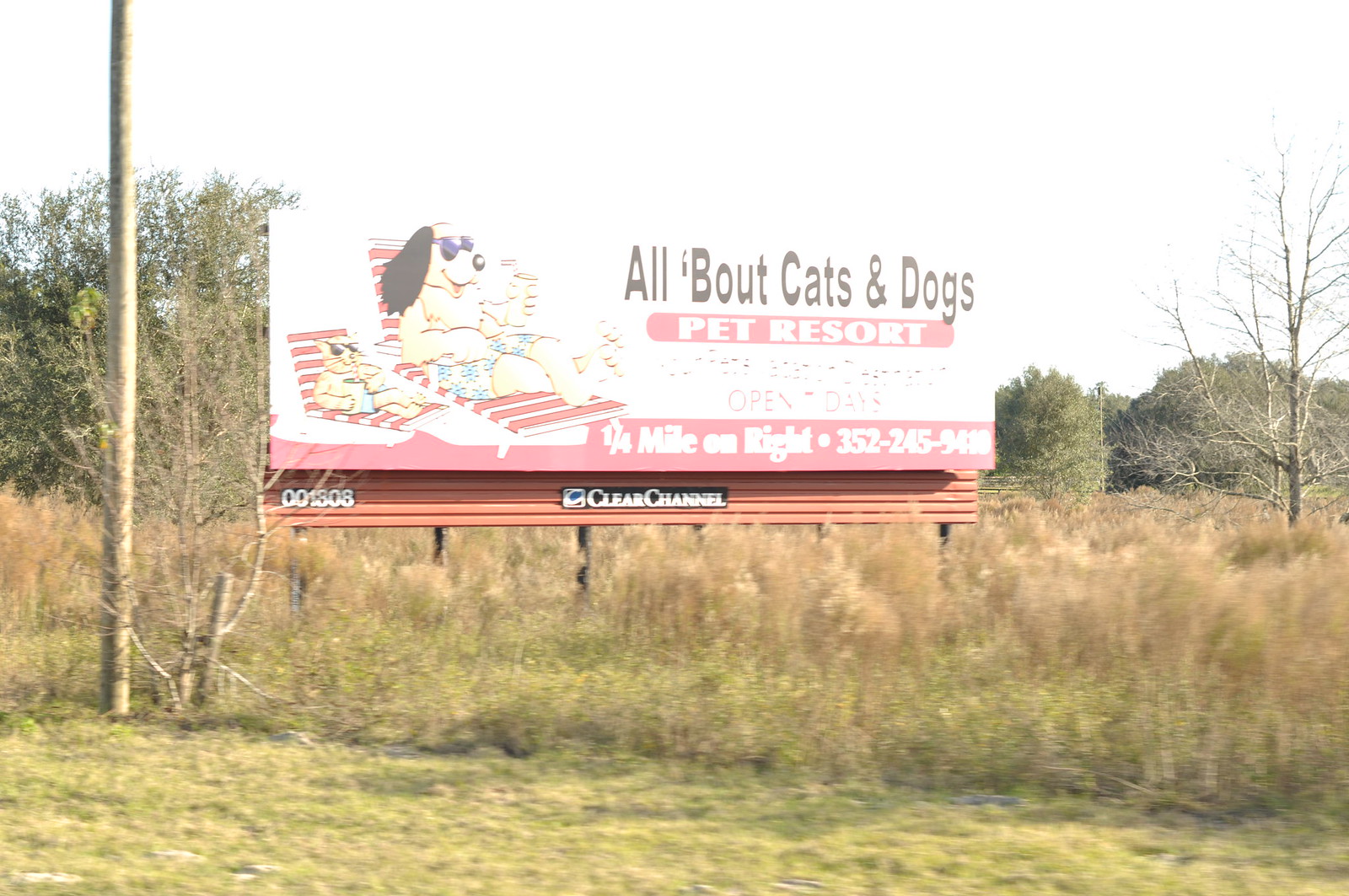This outdoor photograph captures a roadside billboard set against a white sky. The foreground features a mix of green and brown grass, transitioning into taller, bushy vegetation that reaches the base of the billboard. Surrounding the area are some bare trees and denser, leaf-covered trees in the background. To the left, a tall telephone pole can be seen, though its wires remain out of frame. The billboard, marked by the Clear Channel logo, prominently displays an advertisement for the "All About Cats and Dogs Pet Resort." The left side of the sign shows two reclining beach chairs: a smaller one holding a white cat with sunglasses and a larger one occupied by an anthropomorphic yellow dog with black ears, also wearing sunglasses, swim trunks, and holding a beverage. The right side of the billboard includes informative text, "All about Cats and Dogs Pet Resort, open daily, quarter mile on right," followed by a phone number, 352-254-9480. The image appears slightly blurred, suggesting it might have been taken from a moving vehicle.